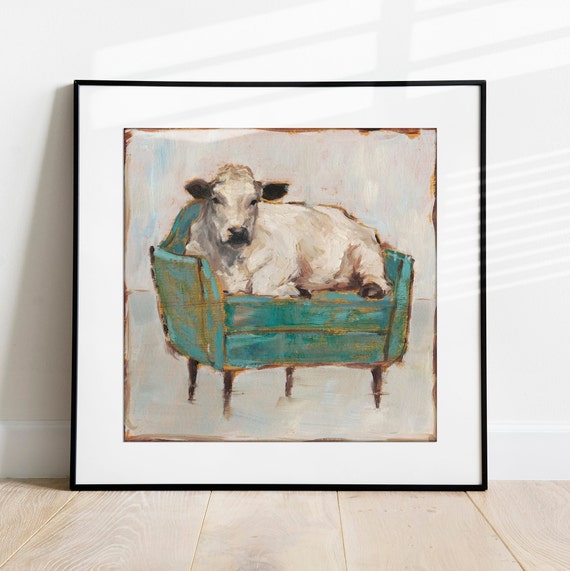This photograph showcases a meticulously framed painting against a white wall, with a white floor visible at the bottom. The painting, enclosed in a thin black frame, beautifully captures a serene scene with a cream background almost blending with the subject – a white calf with black ears, lounging on a turquoise chair akin to the shade of Tiffany's jewelry boxes. The chair, featuring four brown, likely wooden legs, supports the relaxed calf, which has a brown nose and hooves. This visually calming image, possibly created with watercolor, exudes tranquility as it rests on a light pine wood surface. There are no texts within the photograph or the painting itself, enhancing its elegant simplicity and aesthetic appeal.